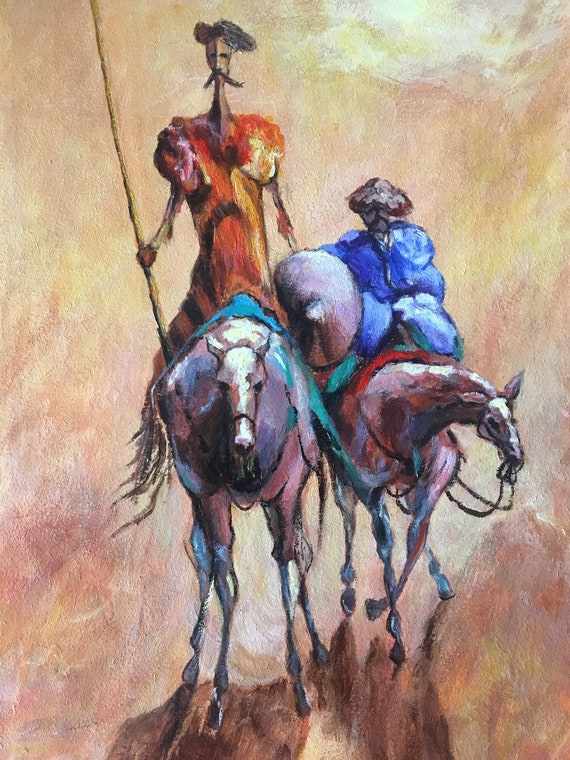The painting showcases a vibrant and dynamic scene set against a richly blended backdrop of yellow and red hues. Central to the composition are two horses, each adorned with colorful blankets instead of visible saddles. The horse in the foreground is in motion, with its foot poised as if mid-step, carrying a distinct figure. This figure is a man dressed in yellow, sporting a long mustache that extends beyond his face. He commands attention with a long yellow staff in his hand and wears a black hat that adds to his imposing presence. The second horse carries what seems to be a blue blob, suggesting it might be laden with belongings rather than a person. The use of bold colors and dynamic posture infuses the image with a sense of movement and narrative intrigue.